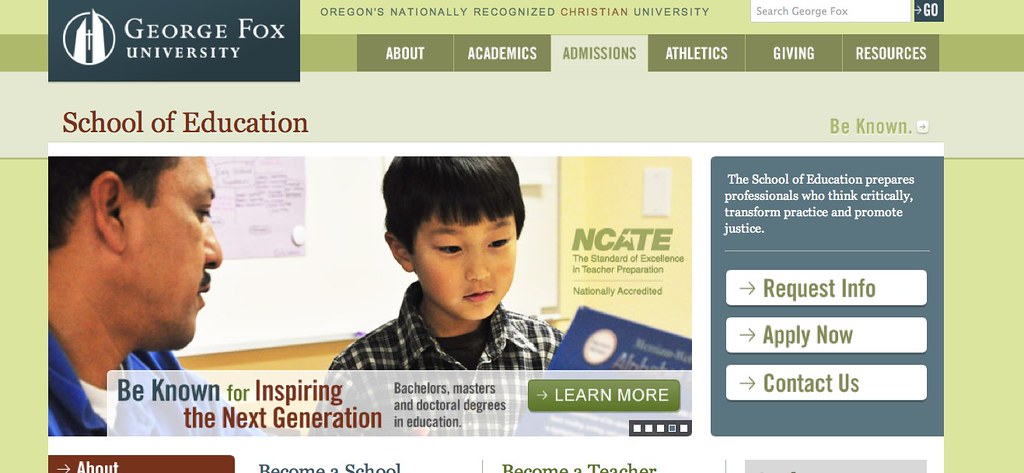This image depicts the homepage of George Forks University, prominently featuring its logo in the top left corner. The text declares the institution as "Oregon's nationally recognized Christian University." A search bar labeled "Search George Forks" is embedded near the top, facilitating easy navigation. Below the search bar are dropdown menus for various sections: "About," "Academics," "Admissions," "Athletics," "Giving," "Resources," and the "School of Education." Additional interactive options are available, including "Request Info," "Apply Now," and "Contact Us." The homepage also champions the university's mission with the slogan "Be Known for Inspiring the Next Generation" and highlights the range of educational programs offered, including bachelor's, master's, and doctoral degrees in education. Calls to action such as "Learn More," "Become a Teacher," and simply "Be Known" emphasize the institution's commitment to shaping influential educators.